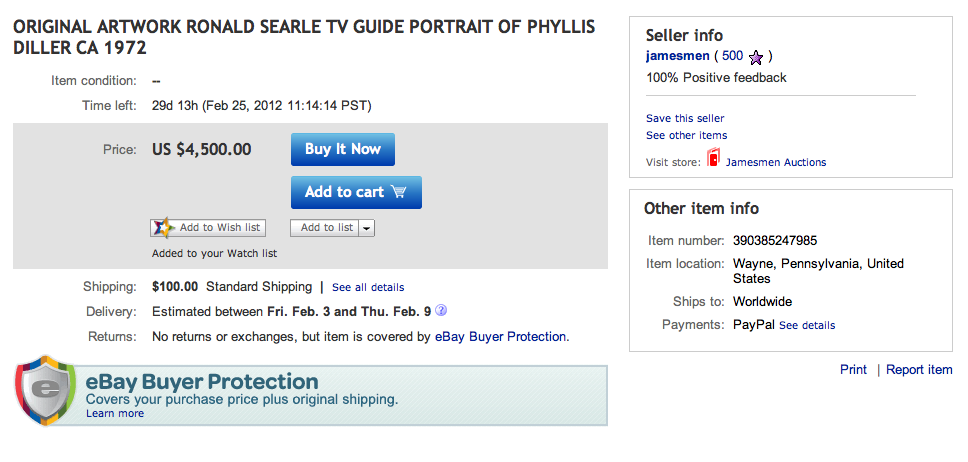eBay Listing for Original Artwork: TV Guide Portrait of Phyllis Diller by Ronald Searle (1972)

This screenshot represents an eBay listing for an original artwork by Ronald Searle, featuring a TV Guide portrait of Phyllis Diller from 1972. The details of the listing are presented in a clear and structured format, predominantly in black, bold, and capital letters across the top of the page.

**Item Details:**
- **Condition:** Not specified 
- **Time Left:** 29 days, 13 hours (as of February 25, 2012, at 11:14:14 Pacific Standard Time)
- **Price:** $4,500
- **Purchase Options:** "Buy It Now" button in blue, and "Add to Cart" option below
- **Wishlist Options:** Includes "Add to Wish List" and "Add to List"

**Shipping Information:**
- **Shipping Cost:** $100
- **Additional Details:** "See all details" link in blue
- **Estimated Delivery:** Between Friday, February 3rd, and Thursday, February 9th
- **Return Policy:** No returns or exchanges, but covered by eBay Buyer Protection

**Protection Services:**
- Icon featuring the eBay symbol on a shield placed on a gray background with the traditional red, blue, yellow, and green colors. The text below states "eBay Buyer Protection covers your purchase price plus original shipping" with a "Learn more" link in a darker greenish-blue color.

**Seller Information:**
- **Seller:** James Man
- **Feedback:** 500 feedbacks, 100% positive
- **Store Name:** James Men’s Auctions
- **Store Icon:** A red door
- **Store Links:** Options to "Save seller," "See other items," or "Visit store" (the latter in black, the others in blue)

**Item Specifics:**
- **Item Number:** Available in the item information section
- **Location:** Wayne, Pennsylvania, United States
- **Worldwide Shipping:** Yes
- **Payment Method:** PayPal
- **Additional Options:** Button to "Print" or "Report" the item

The detailed description encapsulates every aspect of the screenshot, ensuring a potential buyer has all the information needed to make an informed purchase decision.